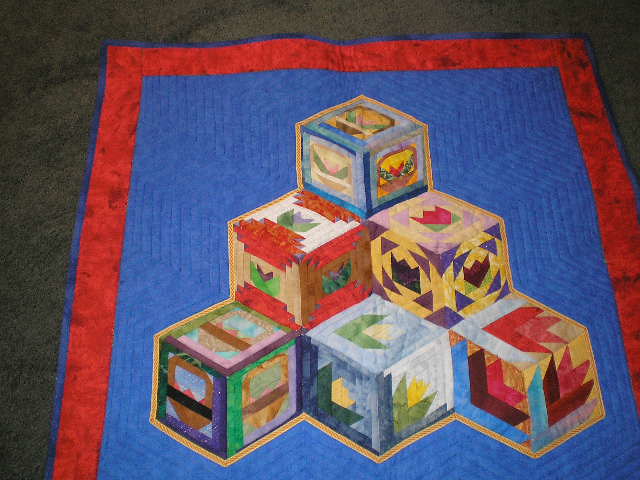The image depicts a detailed photograph of a hand-knit rug situated indoors, likely in someone's home, placed on top of a gray carpet. The rug features a blue border, followed by a thicker bright red border. The main background of the rug is a lighter bright blue color. Central to the design is a series of six three-dimensional cubes arranged in a pyramid formation, reminiscent of the game Qbert. These cubes exhibit a variety of colors including vibrant red, white, purple, yellow, green, blue, and brown, each adorned with intricate and unique patterns such as triangular shapes and possibly tetrahedrons. The topmost cube has blue borders interspersed with various designs, while the other cubes display patterns with red, white, purple, yellow, green, and blue, creating a visually striking and colorful centerpiece against the blue background.